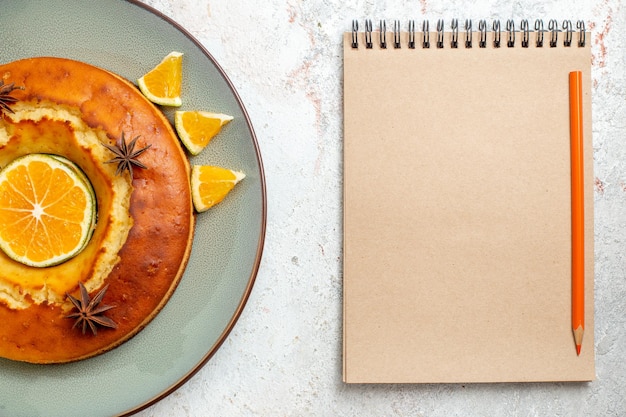In this detailed image, a serene breakfast scene is captured on a marbled countertop, perhaps made of granite. On the right side, there is a cream-colored spiral notepad with a simple orange pencil resting on top, poised for writing but currently untouched. The intricate marbling of the countertop provides a beautiful backdrop for the setting.

To the left of the notepad is a round seafoam green plate with a decorative brown edge. Centered on the plate is a golden-brown pancake, adorned with a large flat slice of orange and three pieces of star anise artfully arranged on top. Additionally, three small, pointed wedges of orange are neatly placed around the pancake, adding to the visual appeal. The combination of the earthy tones of the countertop, the vibrant colors of the plate and food, and the ready-to-use notepad creates a tranquil and inviting breakfast tableau.